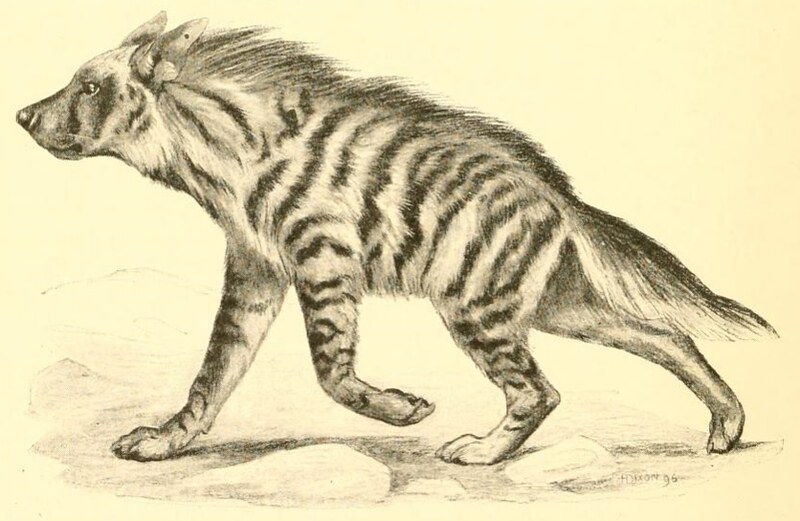The image is a detailed, hand-drawn illustration of an animal that most resembles a hyena with some mixed characteristics of a wolf and a tiger. The animal, facing left, appears to be in motion as if it’s walking forward. It has a white forehead and cheeks, while the rest of the face transitions into darker stripes. The body is predominantly white with black stripes running across it, akin to a tiger's pattern. The animal's head has long, thin ears that stick out to the sides, and its head is lifted with a closed mouth. Its front left paw is off the ground, indicating movement, with similar motion depicted in its back legs. The background is an off-white, cream color, suggesting the paper is old or yellowed with age, enhancing the illustration's classic, scientific feel. Shadows and slight details, such as small rocks on the ground, add depth to the drawing, emphasizing the black and white elements predominantly used.